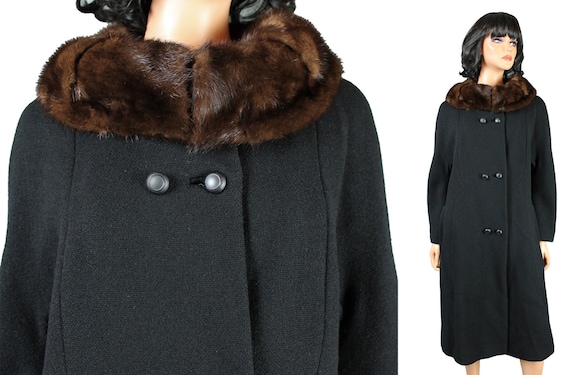The vertical rectangular image features a mannequin modeling a stylish knee-length coat. On the right, the mannequin is shown in full length, revealing the coat that extends just below the knees and reaches down to the wrists. The coat is double-breasted with a total of six goldish buttons arranged in three levels, two buttons at each level. It is a dark color, possibly black, and has a luxurious brown fur collar. The mannequin has shoulder-length black hair with bangs and is gazing upward into the distance. On the left side of the image, there is a close-up showing just the top half of the coat, highlighting the buttons and the fur collar in more detail. The background is plain, ensuring that focus remains solely on the mannequin and the coat.